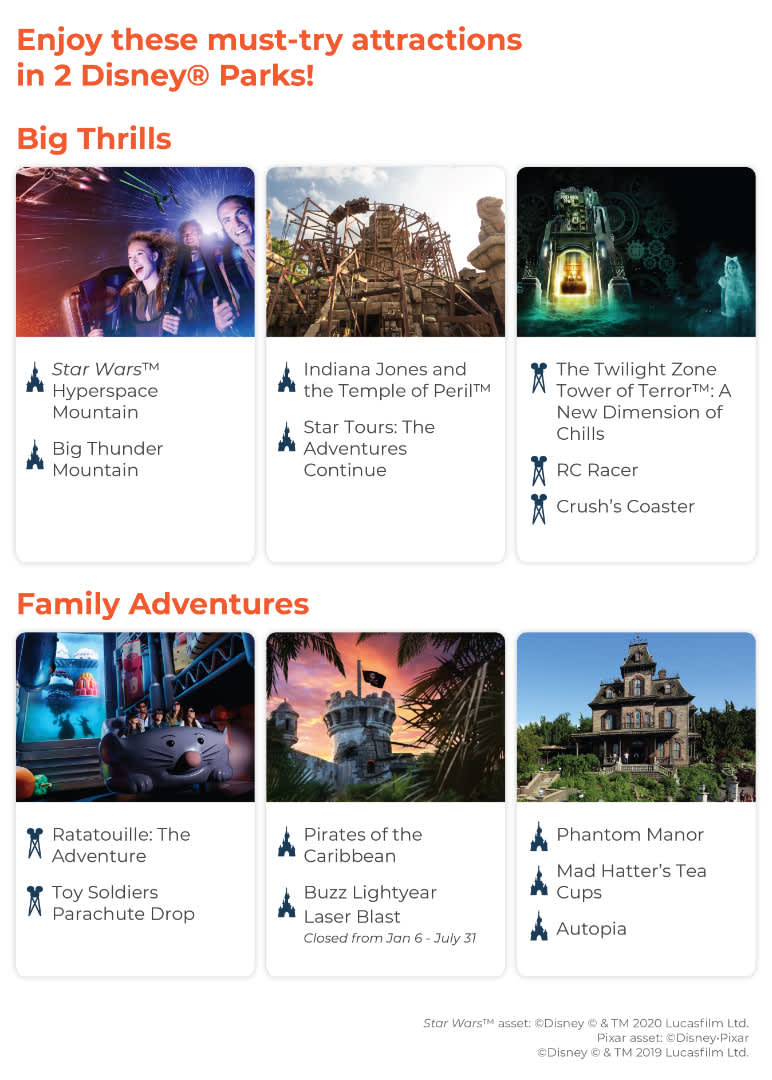This image appears to be a promotional graphic from a Disney parks website, highlighting must-try attractions at two Disney parks. At the top, an orange banner enthusiastically states, "Enjoy these must-try attractions in two Disney parks - big thrills." Below this banner, the image is divided into different sections showcasing various rides along with their respective photographs.

The first row features three images of thrill rides. On the left, there's an image of people screaming on a roller coaster labeled "Star Wars Hyperspace Mountain" and "Big Thunder Mountain." The middle image, depicting a brown structure, is captioned "Indiana Jones and the Temple of Peril" and further highlighted with "Star Tours, the adventure continues" below it. On the right, a dark, eerie photo with green hues showcases "The Twilight Zone Tower of Terror: A New Dimension of Chills," with "RC Racer" and "Crush's Coaster" listed beneath it.

The second section, marked with another orange banner that reads "Family Adventures," presents images geared toward family-friendly experiences. On the left, there's a whimsical picture of a ride resembling a cat or mouse, titled "Ratatouille: The Adventure," followed by "Toy Soldiers Parachute Drop." The central image depicts a castle with a flag and surrounding trees, labeled with "Pirates of the Caribbean" and the playful "Buzz Lightyear Laser Blast" underneath. The rightmost picture, resembling a haunted house, is marked "Phantom Manor," with "Mad Hatter's Teacups" and "Autopia" underneath.

Each ride listed is accompanied by an icon of a pair of scissors on the left side—sometimes the scissors are closed and pointing upward, other times they are open and pointing downward, although the significance of this icon is unclear.

Overall, the image effectively showcases a variety of attractions at Disney parks, enticing visitors with both high-adrenaline and family-friendly options.